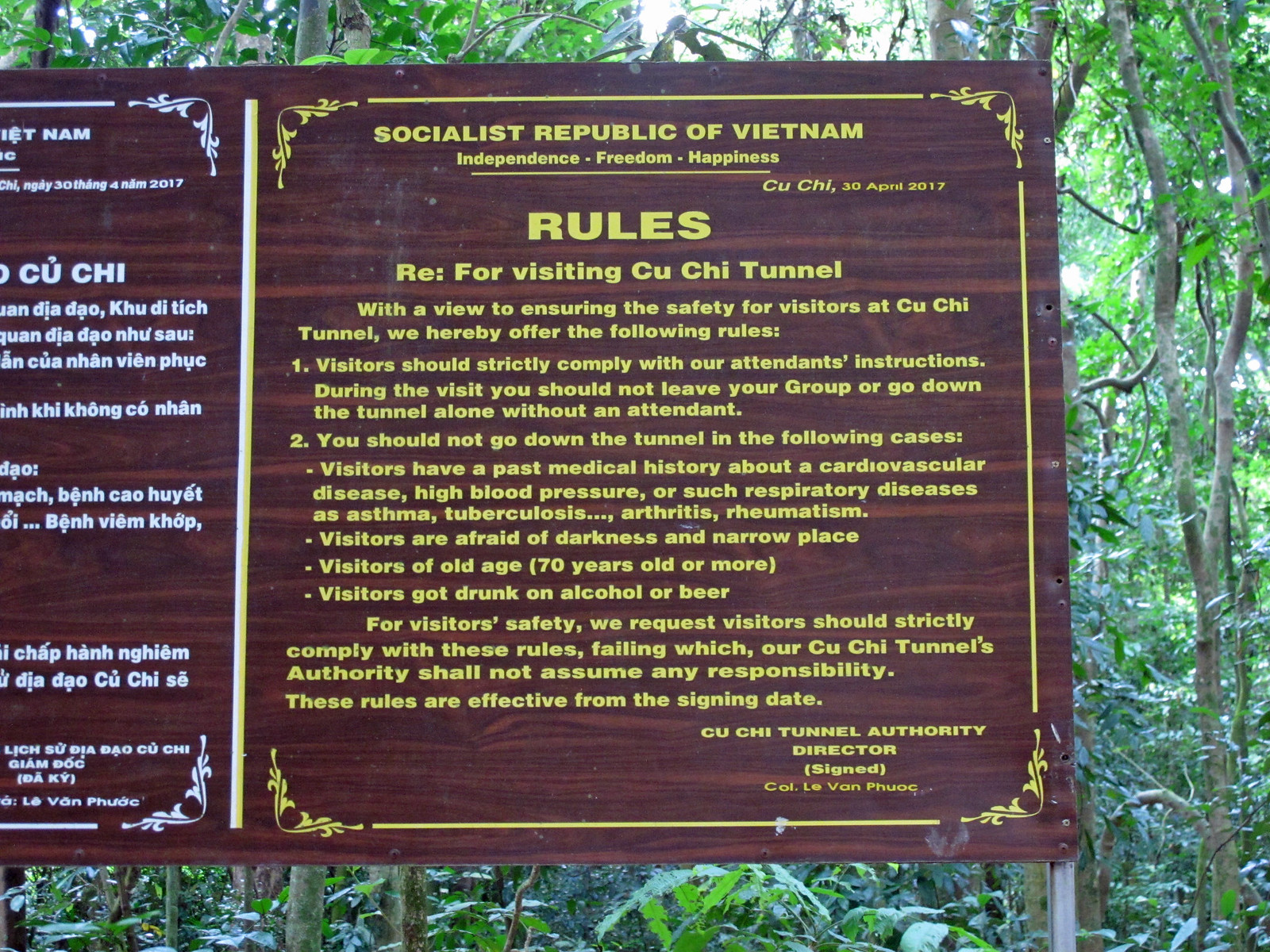The photo depicts a wooden sign situated in a lush, forested area, likely in Vietnam. The background features tall, thin, healthy trees with white bark and green leaves, creating a dense jungle ambiance. The sign itself dominates approximately 70% of the image.

On the left side, the sign appears to be written in Vietnamese with white text. The right side, fully visible and in English with gold text, reads:

"Socialist Republic of Vietnam  
Independence, Freedom, Happiness  
Cu Chi  
30 April 2017

Rules for visiting Cu Chi Tunnel:

1. Visitors must strictly comply with our attendant's instructions. Do not leave your group or enter the tunnel without an attendant.  
2. Entrance to the tunnel is prohibited for visitors with cardiovascular disease, high blood pressure, respiratory conditions like asthma or tuberculosis, arthritis, rheumatism, fear of darkness or narrow spaces, those aged 70 years or older, and anyone under the influence of alcohol or beer.  
3. For visitors' safety, adherence to these rules is mandatory. Non-compliance will result in the Cu Chi Tunnel Authority not assuming any responsibility.

These rules are effective from the signing date.

Signed, Colonel Le Van Phuoc, Cu Chi Tunnel Authority Director."

The sign emphasizes ensuring visitor safety while exploring the Cu Chi Tunnels.